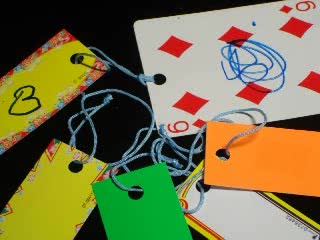This small image features a six of diamonds playing card in the upper right corner, adorned with blue ink scribbling in its center. A hole is punched in the top left of the card, threaded with a blue string that connects to a rectangular yellow label, prominently marked with a black 'B'. Beside this setup, several unattached labels are scattered around. These labels are paper or thin cardboard rectangles in various colors: yellow, green, white, and orange, each with a blue string threaded through a hole at the top. The image presents a quirky and somewhat disordered assortment of labeled cards and tags, with the highlighted six of diamonds playing card serving as the focal point.